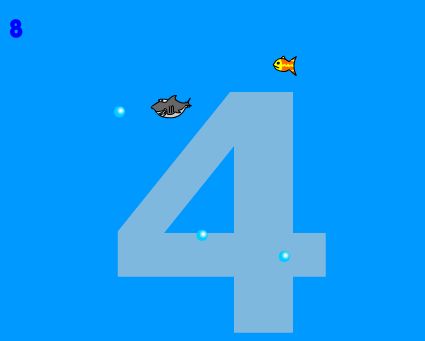The illustration features a digital ocean-themed scene against an aqua blue background. Dominating the composition is a large, off-center greyish-blue number 4 with a looping design. Scattered around the number 4 are several turquoise blue bubbles, each highlighted in white, with one of these bubbles positioned toward the top left.

In the top left corner of the image, a smaller navy blue number 8 stands out against the bright background. Together with this layout, two fish add life to the scene. Above and to the right of the number 4 swims a vibrant yellow and orange fish, while to the left of the number 4, a small, shark-like grey fish with a lighter grey belly appears. The latter, slightly bigger than the goldfish, features a distinct fin on its back. The visual elements — from numbers and bubbles to colorful fish — collectively create a compelling underwater ambiance, suggestive of a video game interface.